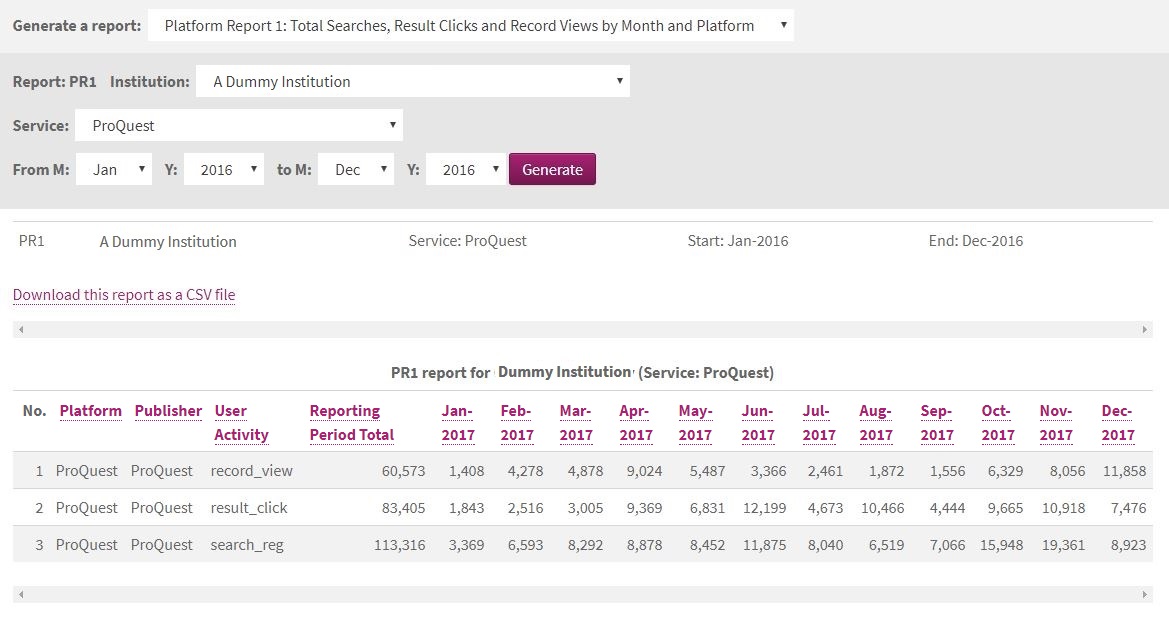Detailed Caption:

The image displays a comprehensive report titled "Texas's January Report: Platform Report One." This report, labeled as PR1, provides detailed analytics on the total searches, results, clicks, and record reads for a dummy institution using the ProQuest service. The data spans from January 2016 to December 2016. A section of the report is highlighted in purple text, prompting users to "Download this report to CSV file." 

A gray bar demarcates different sections of the report, clearly showing the PR1 report for the dummy institution with the service provided by ProQuest. Various metrics are presented, including the total user activity during each reporting period. The periods listed are monthly, from January 2016 through December 2017.

Below the section header, detailed statistics such as record views are enumerated. They include:
- January 2016: 60,523 views
- March 2016: 1,408 views
- April 2016: 4,278 views
- May 2017: 4,878 views
- June 2017: 9,024 views
- July 2017: 5,487 views
- August 2017: 3,366 views
- September 2017: 2,461 views
- October 2017: 1,872 views
- November 2017: 1,556 views
- December 2017: 6,329 views

The final totals for the year 2017 are marked at 8,056 views in November and 11,858 views in December, clearly indicating the fluctuating user activity over the reporting periods.